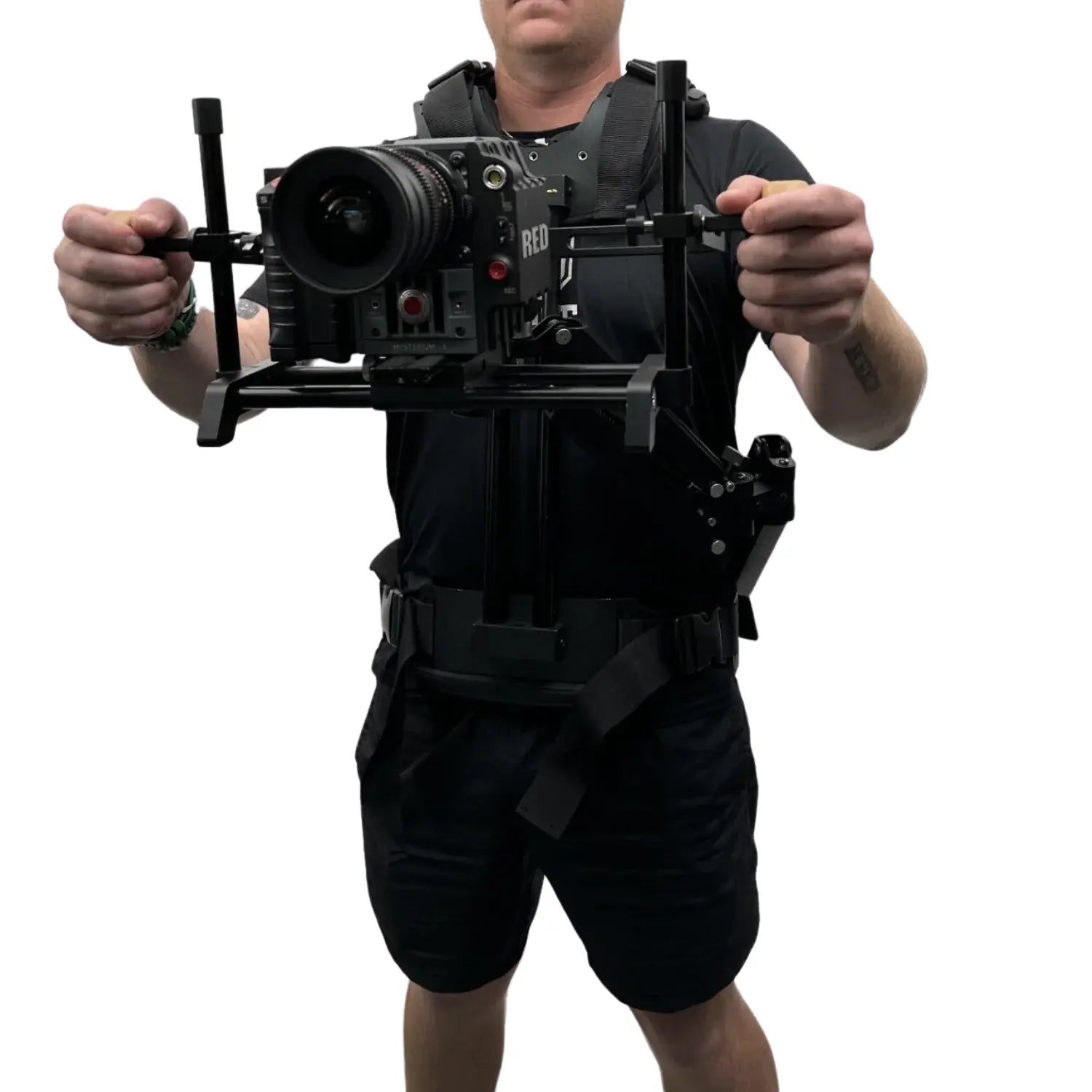In this photograph, a man wearing a black shirt and black shorts is captured from the chest down, his face not fully visible. He is holding a high-tech handheld black camera, which is mounted on an elaborate stabilizing rig. This metal construct is strapped to his body from the waist up, including a thick canvas belt with a large buckle and a vest-like apparatus. The rig extends forward from his waist and chest, allowing the man to support and stabilize the camera with both hands. The camera, affixed to a bar-like shelf on the rig, is angled slightly and features visible knobs. The background of the image is completely white, emphasizing the technical setup.